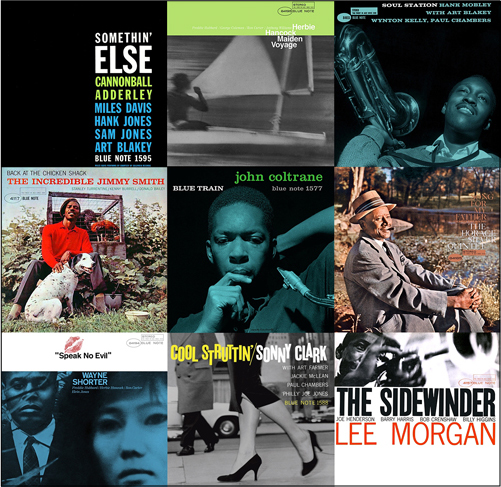The image is a vertical rectangular collage featuring nine jazz album covers arranged in a grid of three rows and three columns. The album covers vary in design, but many share a dark background. Notable inclusions are as follows: 

- The top left cover has a black backdrop with names listed in white, green, and blue text, which include Cannonball Adderley, Miles Davis, Hank Jones, Sam Jones, and Art Blakey.
- The middle cover showcases John Coltrane, with a profile image of him looking down, his hand partially covering his face. It features green lowercase text reading "John Coltrane" with "Blue Note 1577" in italicized white letters below.
- Another cover includes Jimmy Smith, depicted sitting outside while petting a dog, titled "The Incredible Jimmy Smith."
- Other identifiable albums within the collage are “Speak No Evil” by Wayne Shorter, "Cool Struttin'" by Sonny Clark, and "The Sidewinder" by Lee Morgan.
- One cover displays a black man, possibly holding a tuba, rendered with a black background and teal blue text.
- There is also an image of an older black man in a suit, seemingly seated in a park, alongside some difficult-to-read text.

The album covers highlight prominent jazz musicians and incorporate distinctive typography and photography elements, characteristic of jazz album designs.